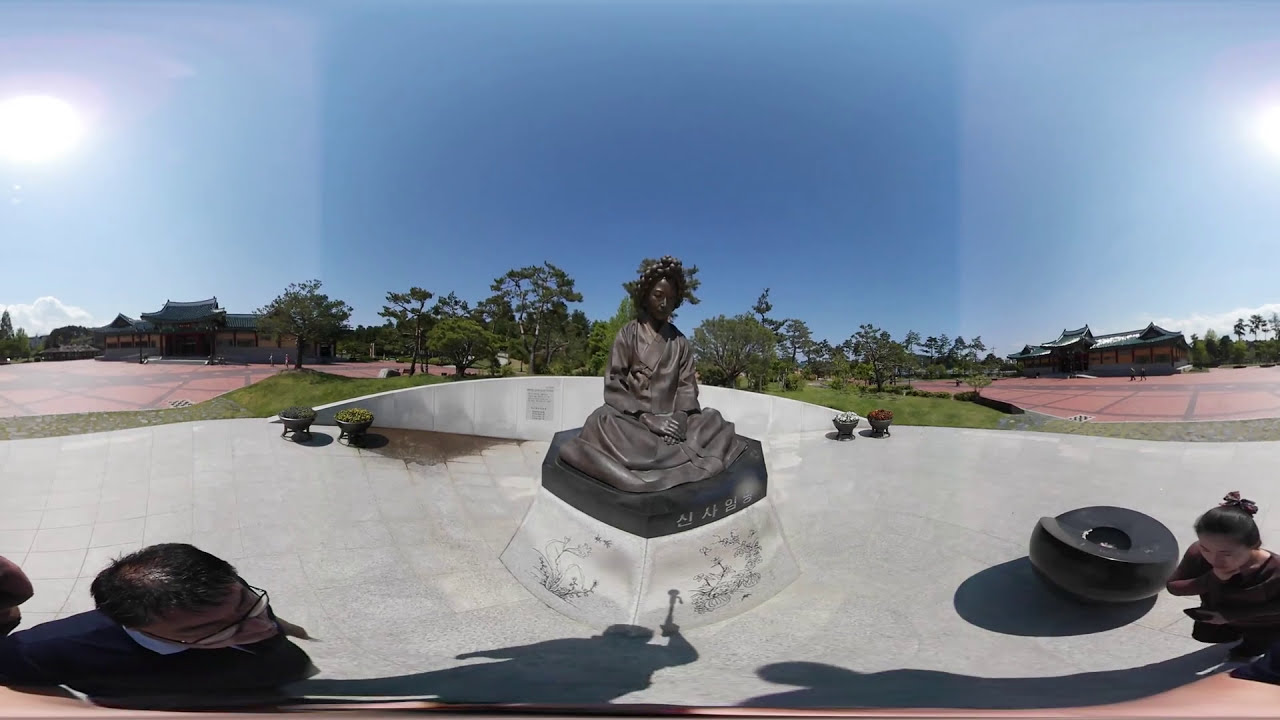This photograph captures a serene sunny day at an outdoor monument featuring a prominently positioned statue on a light-colored concrete platform. The statue, rendered in a bronze or gray stone, depicts a woman donned in a flowing robe, seated with her hands clasped in a prayerful gesture. She wears a decorative crown of leaves or berries on her head and gazes downward in contemplation. The base of the statue, matching the concrete floor, is inscribed with Asian characters—likely Chinese or Japanese.

Two blurred figures, an Asian man in glasses with a blue shirt on the left and a woman with black hair in a reddish shirt or dress on the right, add a dynamic element to the scene as they walk by. The background reveals a blend of traditional Asian architecture, hinting at a possible monastery or heritage site, with structures adorned in reds and greens and featuring distinctive rooflines. Trees, including a notable bonsai, line the background, softened by the clear blue sky. This richly detailed setting suggests the statue serves as a sacred or historic marker within a tranquil courtyard area, inviting visitors for contemplation and reflection.